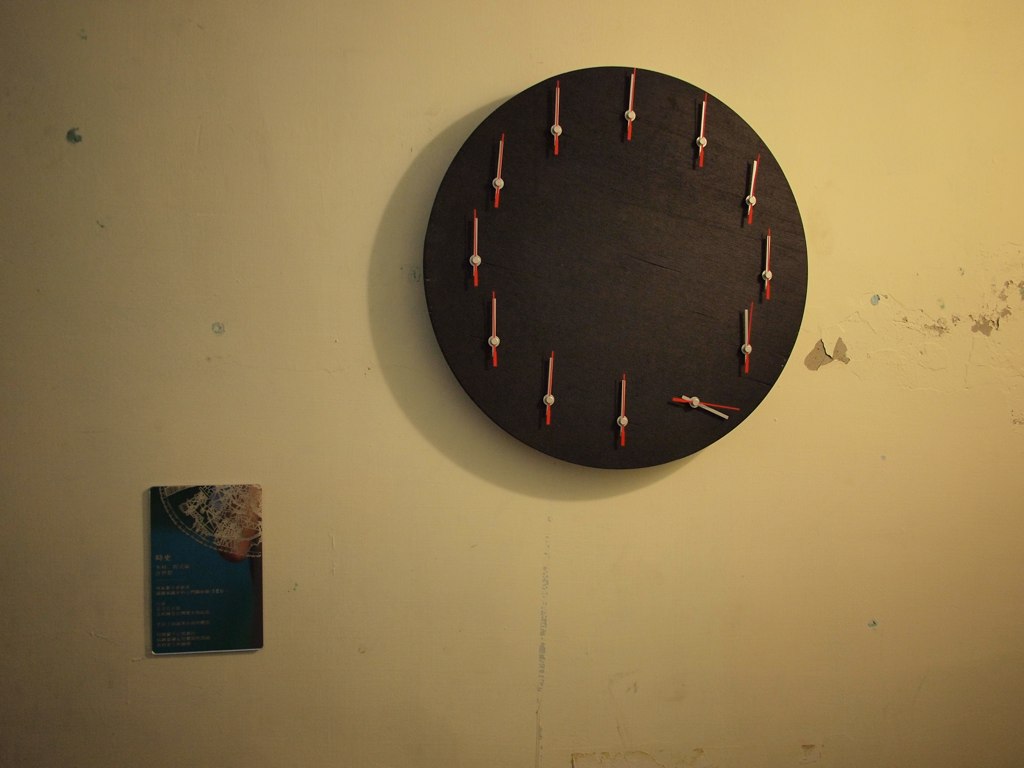The image features a prominent dark brown wooden clock mounted on a distressed cream-colored wall. This unconventional clock has 12 points around its perimeter, each point comprised of minute and hour hands colored in white and reddish-orange. Notably, the hands at the five o'clock position are tilted, pointing towards the right side of the image, unlike the others, which all point upwards. The wall behind the clock is marred with imperfections and peeling paint. In the bottom left corner of the image, there is a rectangular plaque or picture with a dark gradient from black to blue, featuring Asian writing and a unique design, possibly including a woman's elbow.